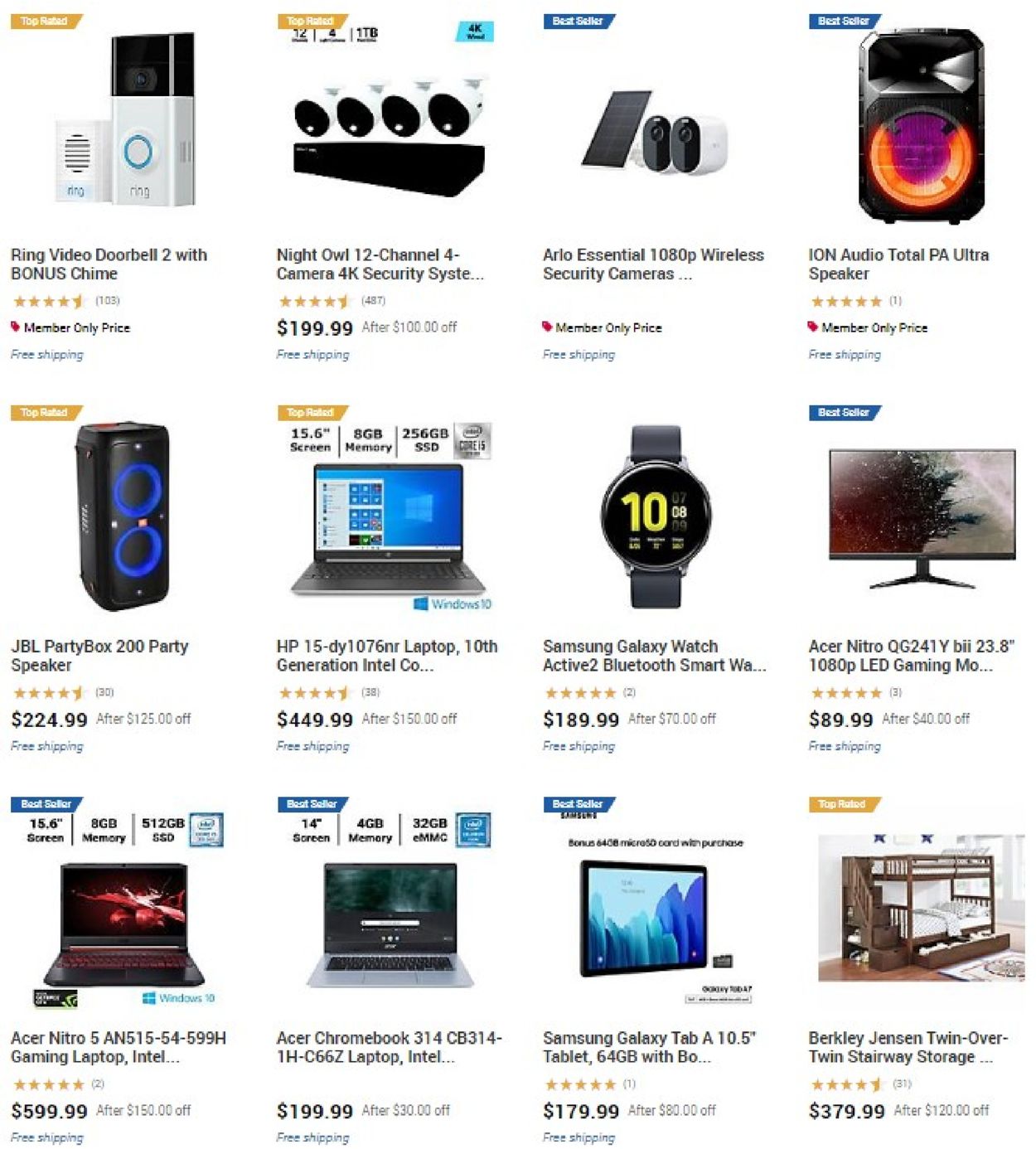### Image Caption: Detailed Description of Search Results Page

The image depicts a search results page organized into three horizontal rows, each row containing four items in a grid format. 

- **First Row, First Item:**  
  - **Product:** Ring Video Doorbell 2 with Bonus Chime
  - **Top Left Corner:** "Top Rated" in light-colored font on a gold rectangular background
  - **Image:** Visual depiction of the Ring Video Doorbell 2
  - **Stars:** 4.5 stars displayed in gold
  - **Reviews:** The number of reviews is in parentheses but too small to read
  - **Price:** "Members Only Price" in black font, with a small red detail next to it
  - **Shipping:** "Free shipping" in blue font
  
- **First Row, Second Item:**  
  - **Product:** Night Owl 12 Channel 4 Camera 4K Security System
  - **Price:** $199.99
  
- **First Row, Third Item:**  
  - **Product:** Arlo Essential 1080p Wireless Security Camera
  - **Price:** Not listed
  
- **First Row, Fourth Item:**  
  - **Product:** ION Audio Total PA Ultra Speaker
  - **Price:** Not listed
  
Each product in the first row features an image positioned above the descriptive text.

- **Second Row, First Item:**  
  - **Product:** JBL Party Box 200 Party Speaker
  - **Stars:** Number of stars displayed under the product title
  - **Price:** $224.99
  - **Shipping:** "Free shipping" noted under the price
  - **Image:** Visual depiction of the JBL Party Box 200 Speaker
  
The layout and information continue in the same structured manner for the rest of the items in the second and third rows, with each product image accompanied by the product name, rating, price if available, and shipping information.